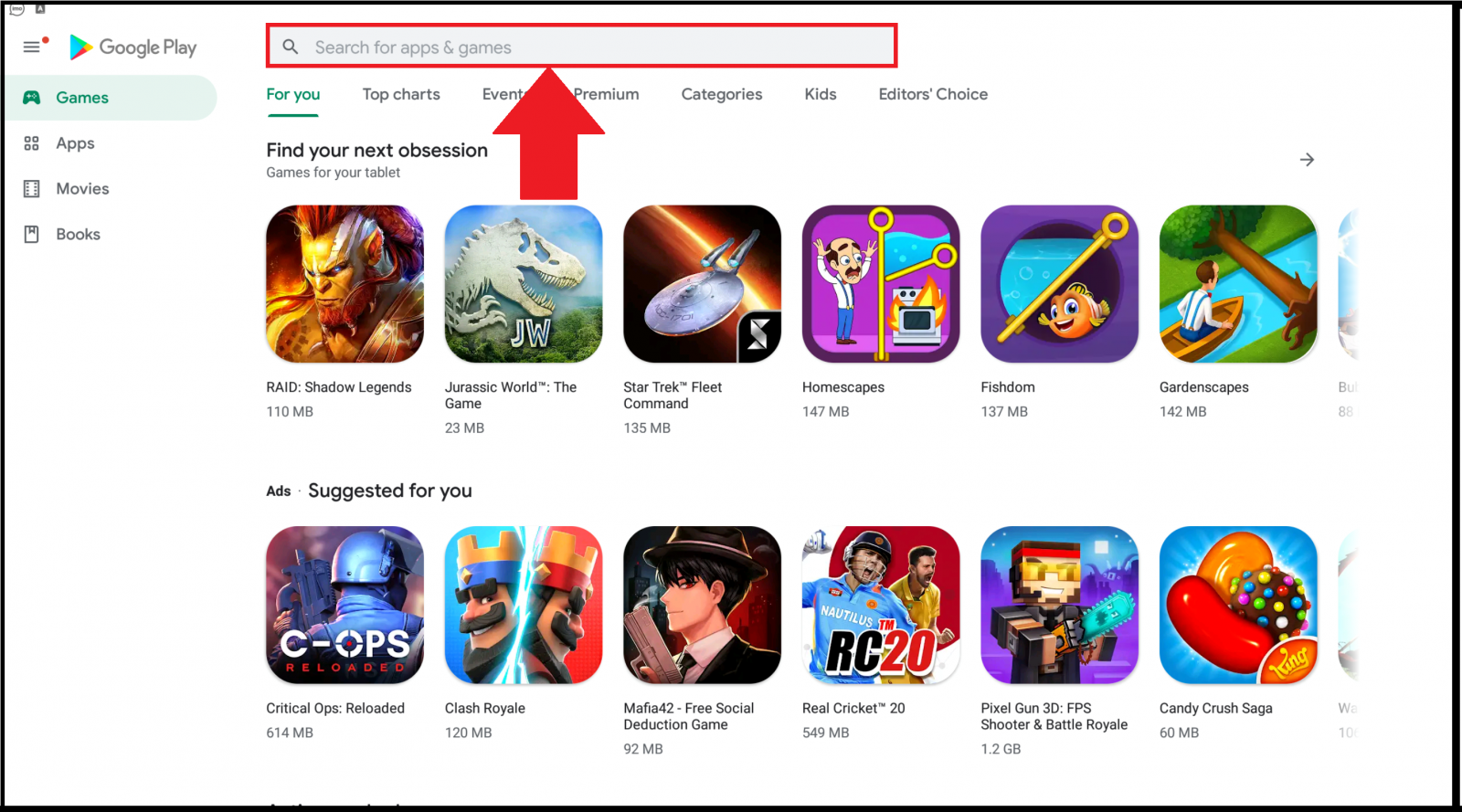A screen capture of a tutorial demonstrating how to search for apps on Google Play Store. The interface is displayed in landscape mode on a mobile device. A red rectangle outlines the search bar, with an arrow pointing to it, and accompanying text indicating, "This is where you would type what you're looking for." Below the search bar, the suggestion "Find your next obsession" is visible, followed by a selection of recommended apps. The first app shows a monstrous figure with the title "Raid: Shadow Legends." The second app features an image of a dinosaur with the initials 'JW' and is titled "Jurassic World: The Game." The third app, "Star Trek Fleet Command," displays a spaceship in space. The fourth app appears to be "Homescapes," depicting a person with a stove on fire. Another app, partially visible, seems to include fish and is associated with "Gardenscapes."